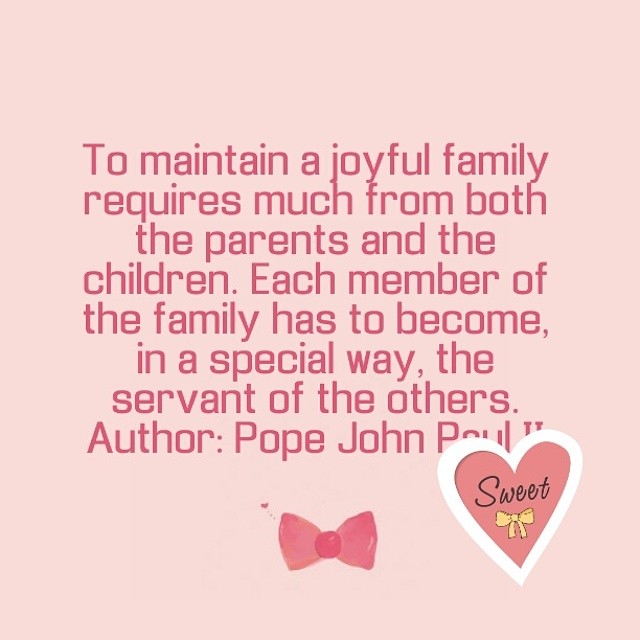The image features a light pink background adorned with various words and pictures. At the center, a quote in darker pink text reads, "To maintain a joyful family requires much from both the parents and the children. Each member of the family has to become, in a special way, the servant of the others." This quote is attributed to Pope John Paul II. Beneath the quote, there is a small pink bow tie, from which a few tiny dots lead to a miniature pink heart. On the bottom right of the image is a heart-shaped sticker with a white border, pink interior, and black text that says "sweet." Beneath the word "sweet" within the heart, there is a small yellow ribbon. The entire composition is set against a light pink square background.